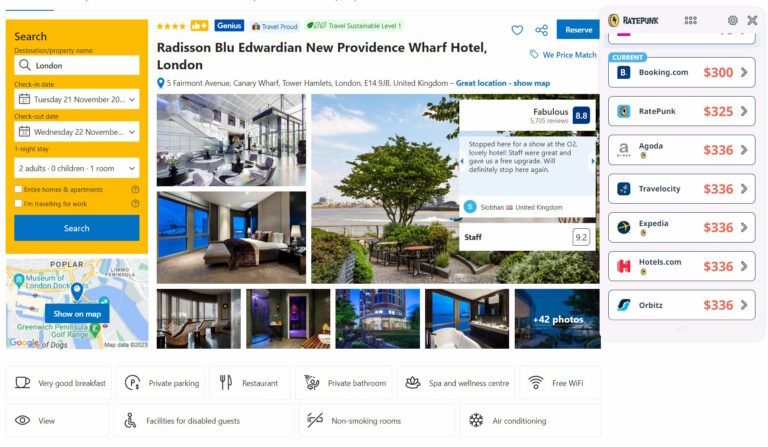This is a screenshot of the Radisson Blu Edwardian, New Providence Wharf Hotel website in London. The central portion of the page displays eight images showcasing various aspects of the hotel, including outdoor views with trees and cozy interiors featuring well-appointed rooms with comfortable beds. Displayed on a yellow background to the left of the images is a search bar. It specifies the location as London and includes date fields for check-in and check-out: Tuesday, November 21st, and Wednesday, November 22nd, although part of the latter date is cut off. It also indicates a booking for 2 adults, 0 children, and 1 room, with the search button highlighted in blue. At the top of the page, the hotel is rated 4 stars, denoted by yellow star icons.